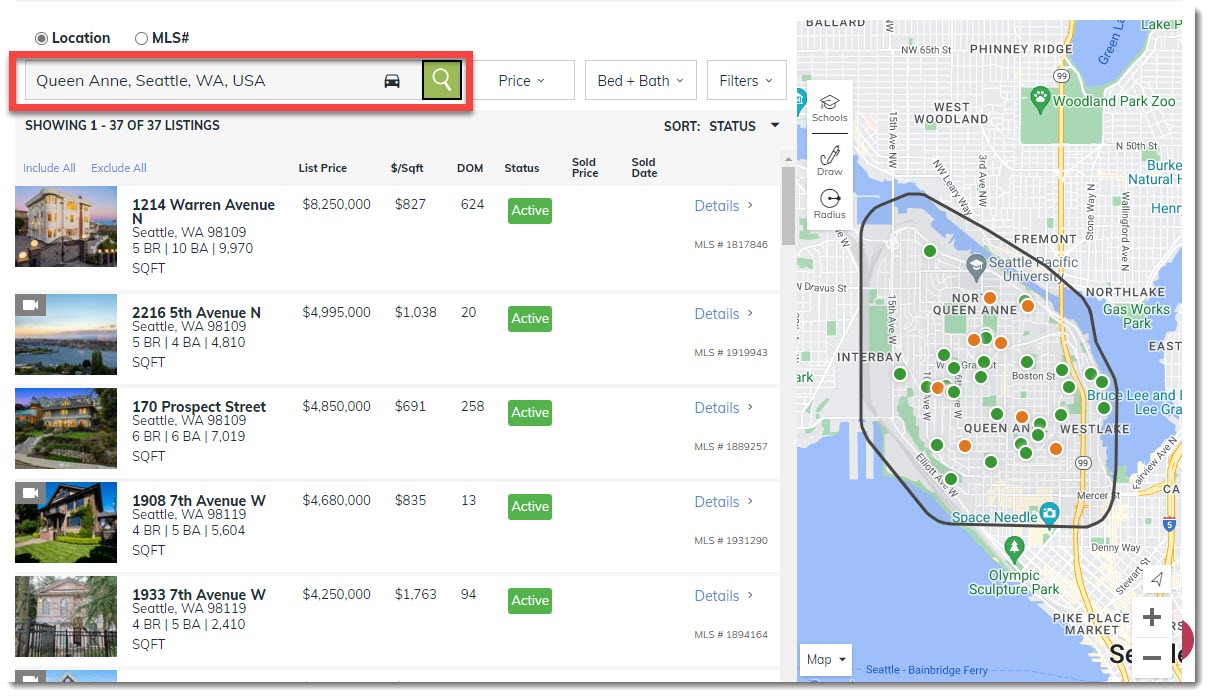The image depicts a real estate listings webpage, characterized by a clean, white background. In the upper left-hand corner are two options for search criteria: "Location," which is selected (indicated by a gray dot in the circle), and "MLS Number," which remains unselected. Below these options is a search bar with the query "Queen Anne, Seattle, Washington, USA." This search bar is flanked by icons: a car icon to the left and a green search button with a red border to the right.

To the right of the search bar are additional filter options: "Price," "Bed and Bath," and "Filters." Directly underneath, the text indicates "Showing 1 of 37 listings." To its right, there's a "Sort Status" option.

Below this header area, there are options to "Include All" or "Exclude All" listings, followed by a table with at least six columns: "List Price," "Price per Square Foot," "DOM" (Days on Market), "Status," "Sold Price," and "Sold Date."

The first row features an image of a building with the following details:  
- **Address:** 1214 Warren Avenue, Seattle, Washington, 98109  
- **Details:** 5 bedrooms, 10 bathrooms, 9,970 square feet  
- **List Price:** $8,250,000 ($827 per square foot)  
- **DOM:** 624 days  
- **Status:** Archived (indicated by a green box)  
- **MLS Number:** 1817846 (small and hard to read)

The second row displays another property:  
- **Address:** 2216 5th Avenue, Seattle, Washington, 98109  
- **Details:** 5 bedrooms, 4 bathrooms, 4,810 square feet  
- **List Price:** $4,995,000 ($1,038 per square foot)  
- **DOM:** 20 days  
- **Status:** Active (indicated by a green box)  
- **MLS Number:** 1919043 (possibly)

The third row shows an illuminated large home with a driveway:  
- **Address:** 170 Prospect Street, Seattle, Washington, 98109  
- **Details:** 6 bedrooms, 6 bathrooms, 7,019 square feet  
- **List Price:** $4,850,000 ($690 per square foot)  
- **DOM:** 258 days  
- **Status:** Active (indicated by a green box)  
- **MLS Number:** 1889257

The fourth row features a home with a green front lawn and two stories:  
- **Address:** 1908 7th Avenue W, Seattle, Washington, 98109  
- **Details:** 4 bedrooms, 5 bathrooms, 5,674 square feet  
- **List Price:** $4,680,000 ($835 per square foot)  
- **DOM:** 13 days  
- **Status:** Active (indicated by a green box)  
- **MLS Number:** 1931790

The final row shows a two-story house behind a black iron gate with a mossy tree in the image:  
- **Address:** 1933 7th Avenue W, Seattle, Washington, 98119  
- **Details:** 4 bedrooms, 5 bathrooms, 2,410 square feet  
- **List Price:** $4,250,000 ($1,763 per square foot)  
- **DOM:** 94 days  
- **Status:** Active (indicated by a green box)  
- **MLS Number:** 1894164

To the image's right side is a map, showing gray land areas and a body of water. The map includes zoom in/out buttons and icons for schools, drawing, and radius. A drawn radius highlights the region encompassing North Queen Anne, part of Interbay, Queen Anne, and Westlake, dotted with numerous green and red indicators.